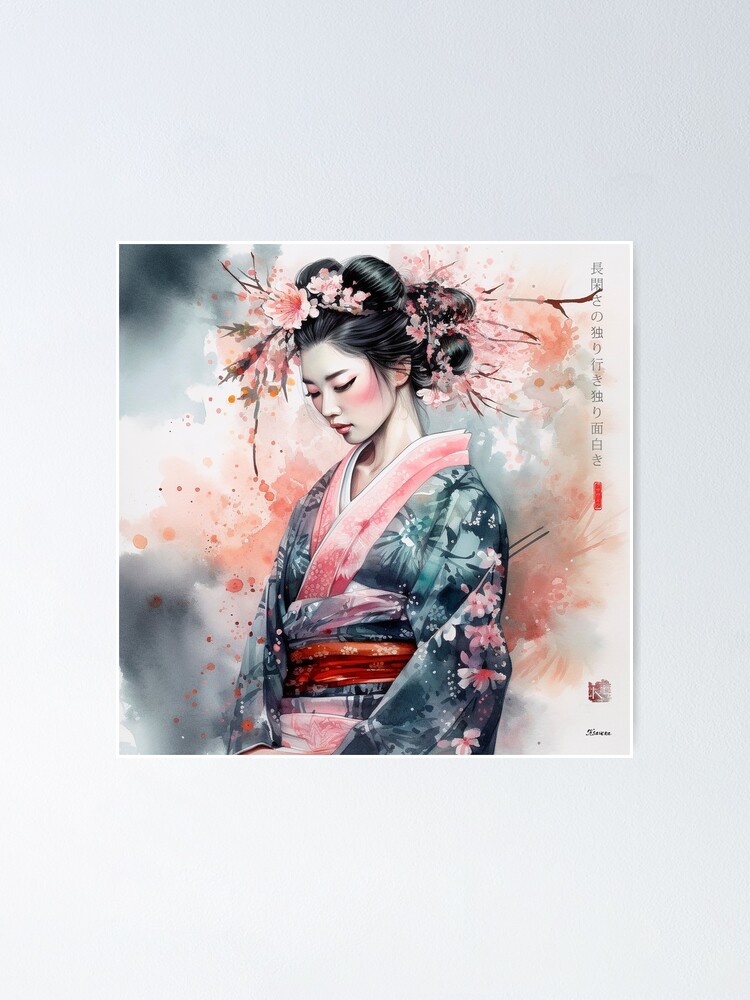This illustration portrays a stylized, modern depiction of a woman, possibly a geisha, dressed in an elaborate kimono. The scene is rendered in a comic illustration style rather than an authentic portrait, underlined by a palette of muted grays and vibrant pinks. The woman, seated alone with her head bowed in apparent thought or meditation, exudes a serene and introspective demeanor. She wears a detailed ceremonial kimono adorned with a motif of sakura blossoms, featuring a harmonious blend of blue, pink, green, and red hues. The kimono, trimmed in pink, has a distinct red obi, matching the blossoms scattered across the fabric. Her hair, jet black and styled into four buns, is decorated with pink-blossomed flowers, echoing the kimono’s floral embellishments. Her porcelain white skin is accentuated with rosy pink cheeks and pink lipstick, while her black eyelashes and eyebrows frame her downcast eyes, adding a sense of quiet elegance to the scene.